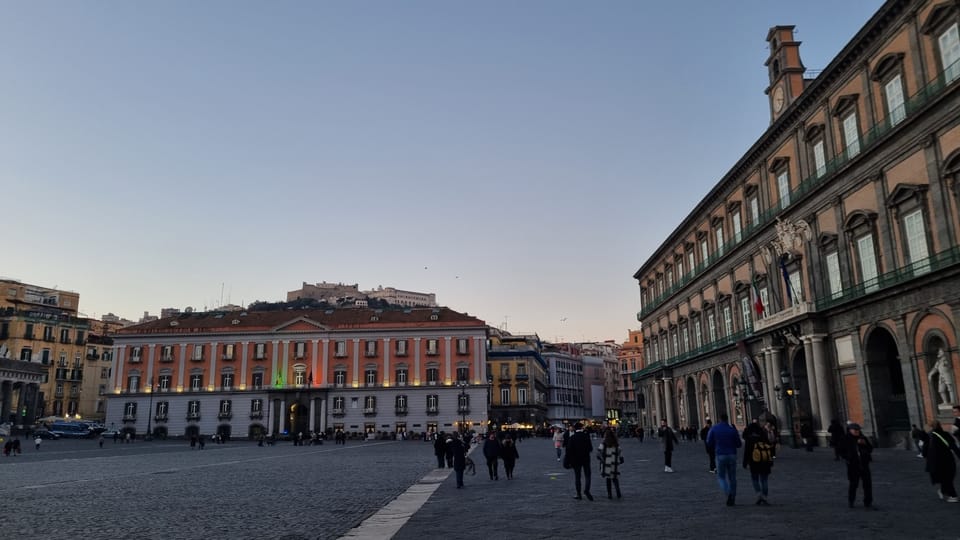The image is a color photograph taken in landscape orientation at sunset, capturing an outdoor scene with a European architectural ambiance. In the middle and to the right of the image stands a grand, historic three-story building with a beige stucco exterior. This building has a series of arches on the ground floor, interspersed with gray statues, and features numerous windows on the upper floors, each adorned with small black-fenced balconies. The second floor has a central, more prominent balcony with a white fence. A clock tower crowns the building, adding to its grandiosity. 

Adjacent and slightly to the left, another three-story building is visible. This structure is distinctive with its pink and white color scheme, featuring long white columns flanking a gabled entrance. Both buildings exhibit classical architectural elements reminiscent of European train stations or tourist attractions, giving off a historical vibe.

The scene is bustling with people walking around a paved square or plaza that lies between these buildings, suggesting a lively public space. The overall atmosphere is vibrant yet historical, with the blue sky tinged pink at the horizon adding a picturesque backdrop. In the distance, a hill with a few structures atop can be seen, enhancing the depth and setting of the image. This photograph represents a realistic portrayal of the Royal Palace of Naples and its surroundings.